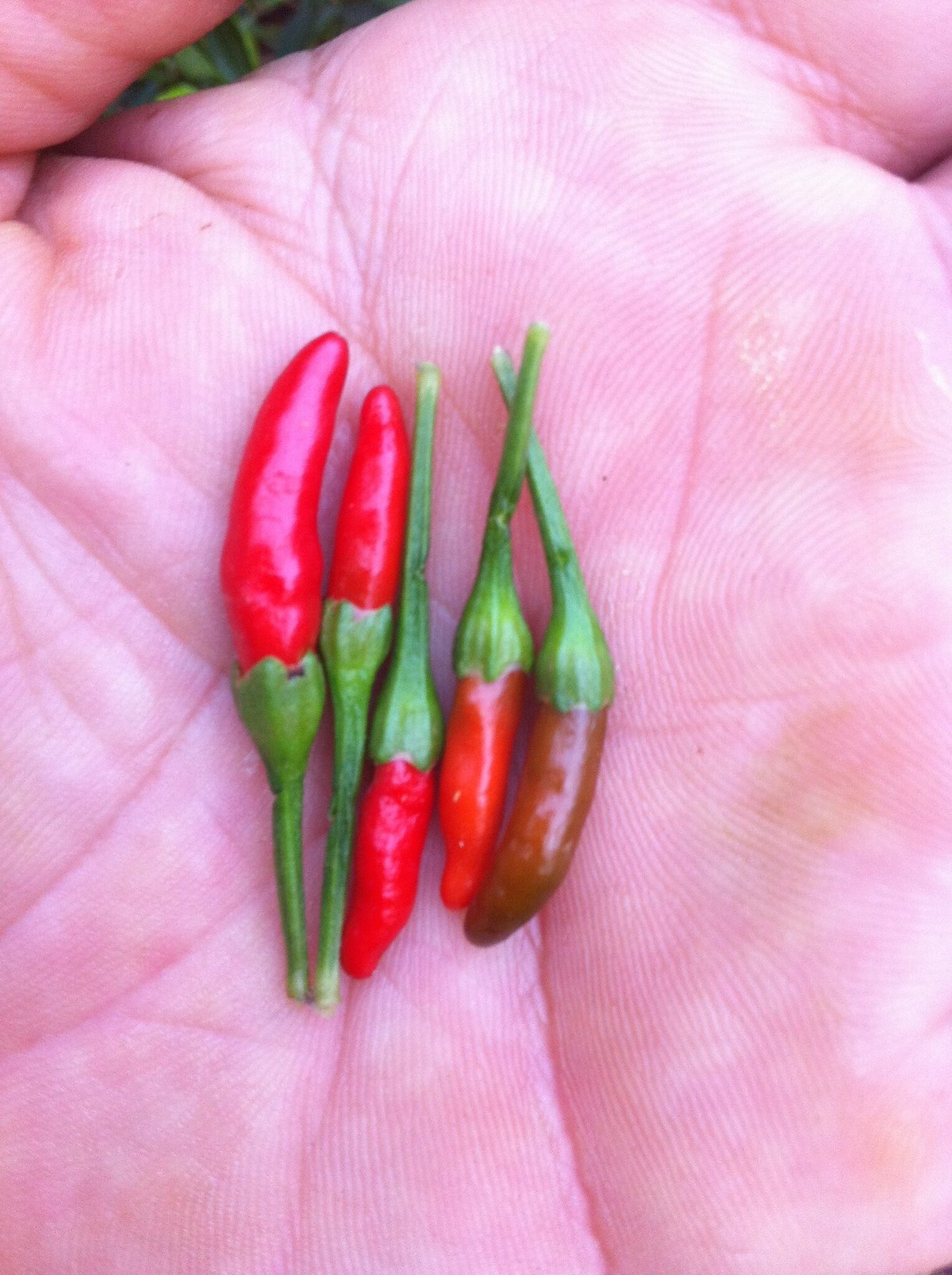The image is a high-resolution, vertical rectangle photograph depicting the palm of a person's left hand held palm-up. The skin is light-colored, and the intricate details of the fingerprints are clearly visible. In the center of the hand’s palm lie five small chili peppers, which are suggested to be Pippin chilies. Each pepper has a vibrant, narrow, curved red tip and a thin green stem, longer than the pepper itself. The two chilies on the left side point upward near the thumb, while the three on the right side point downward. Notably, the pepper farthest to the right has a darker, almost brownish hue, unlike the bright red of the others. The arrangement of the peppers, with precise color details and direction, showcases their small size, collectively fitting into the center of the palm, covering only about half of it.